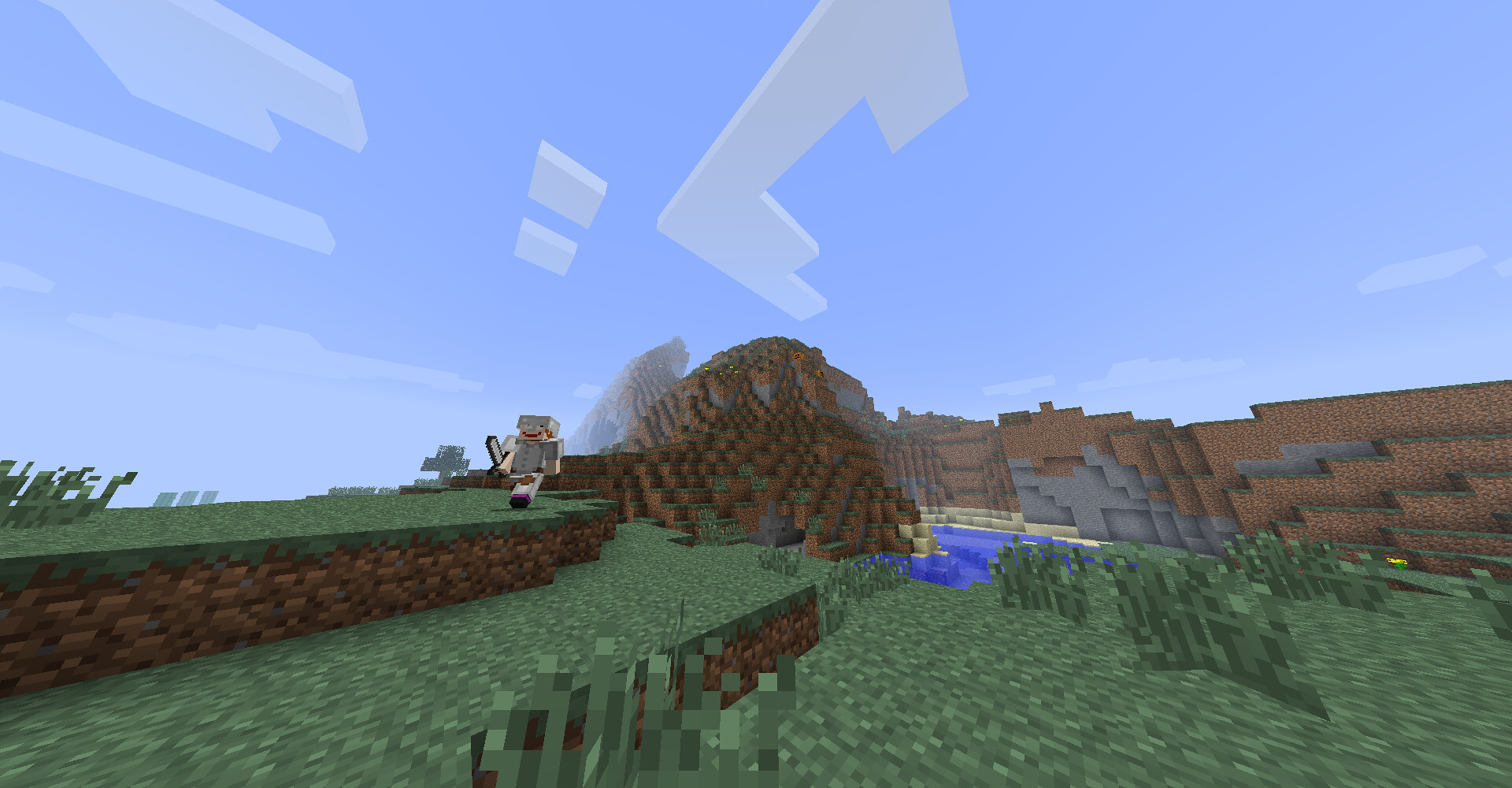In this vibrant still from a video game, the central character stands out with a distinct square head, topped by a gray hat. His facial features are simplified, with a striking red smile that adds to his animated expression. His body is blocky and gray, perfectly in line with the game's geometric aesthetic. His arms, extending outwards, are a peach color, contrasting starkly with the rest of his attire. He wears white pants, accentuated by a purple trim around the ankles, and finishes his ensemble with black shoes.

The character is depicted striding on a terrain that simulates grass, with varying elevations created using stone ledges. Each level of green grass is interspersed with these stone formations, contributing to a dynamic landscape. The background is filled with a serene blue sky dotted with white clouds. To the right, another platform, resembling a brick wall, protrudes into the scene, capped with greenery. Below this section lies a shimmering body of water, adding an element of tranquility to the otherwise structured environment. The overall composition creates a vivid, engaging scene characteristic of detailed video game design.